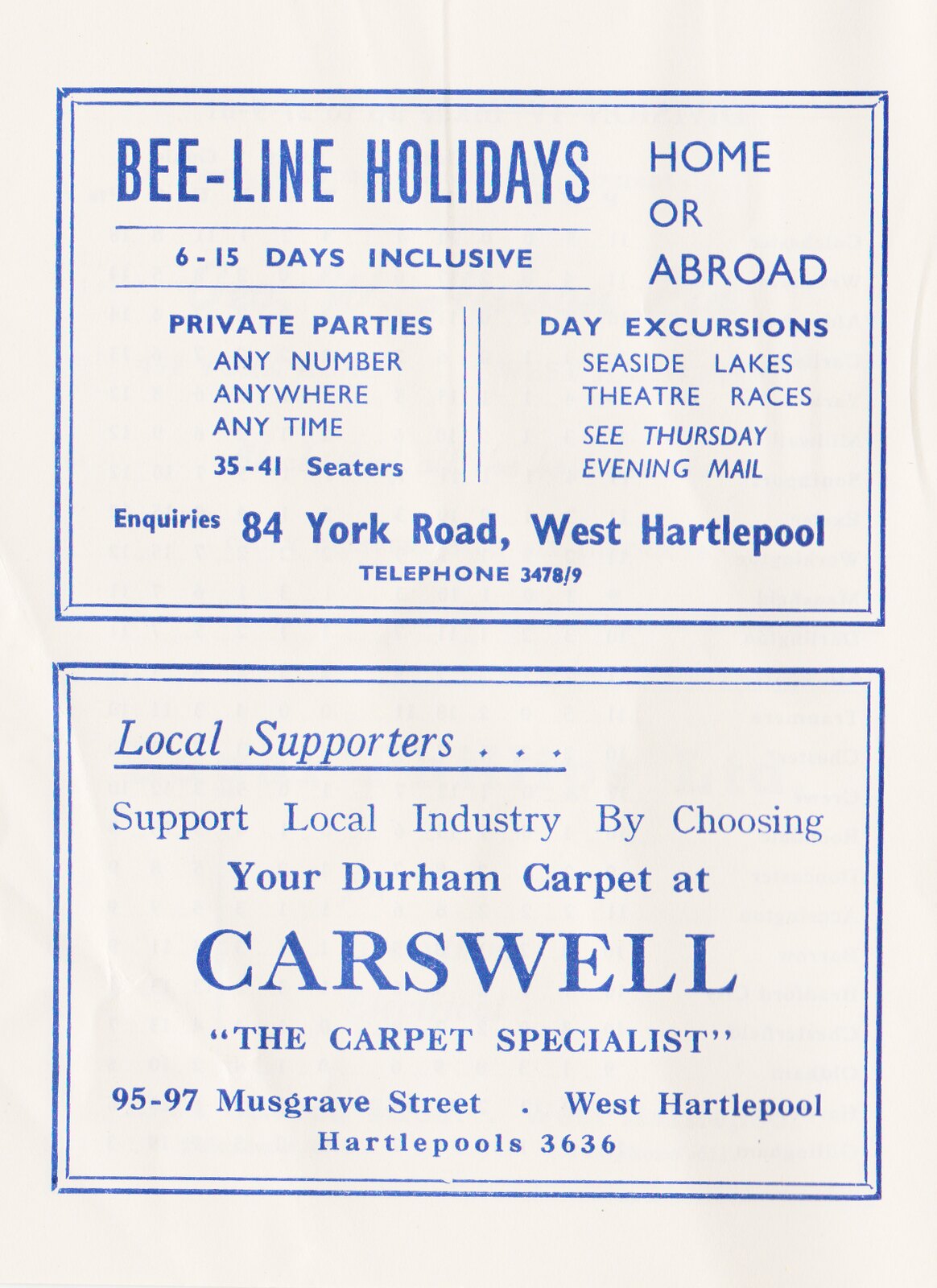The image depicts a white flyer, featuring two distinct advertisements arranged in blue ink. The top advertisement, underlined by the headline "B-Line HOLIDAYS," promotes private parties and excursions ranging from 6 to 15 days, available either domestically or internationally. It caters to groups of any size and offers a variety of outings such as day excursions to seaside locations, lakes, theaters, and races. The contact address for inquiries is 84 New York Road, West Hartlepool, and a telephone number is provided, though it is partially illegible. 

The bottom advertisement, headlined "LOCAL SUPPORTERS," encourages the support of local industries by purchasing Durham carpets from Carswell, the carpet specialist. The address of Carswell is listed as 95-97 Musgrave Street, West Hartlepool, with a contact number provided as Hartlepool 3636. Both sections are set on a white background, with all text rendered in a clear, light blue font.